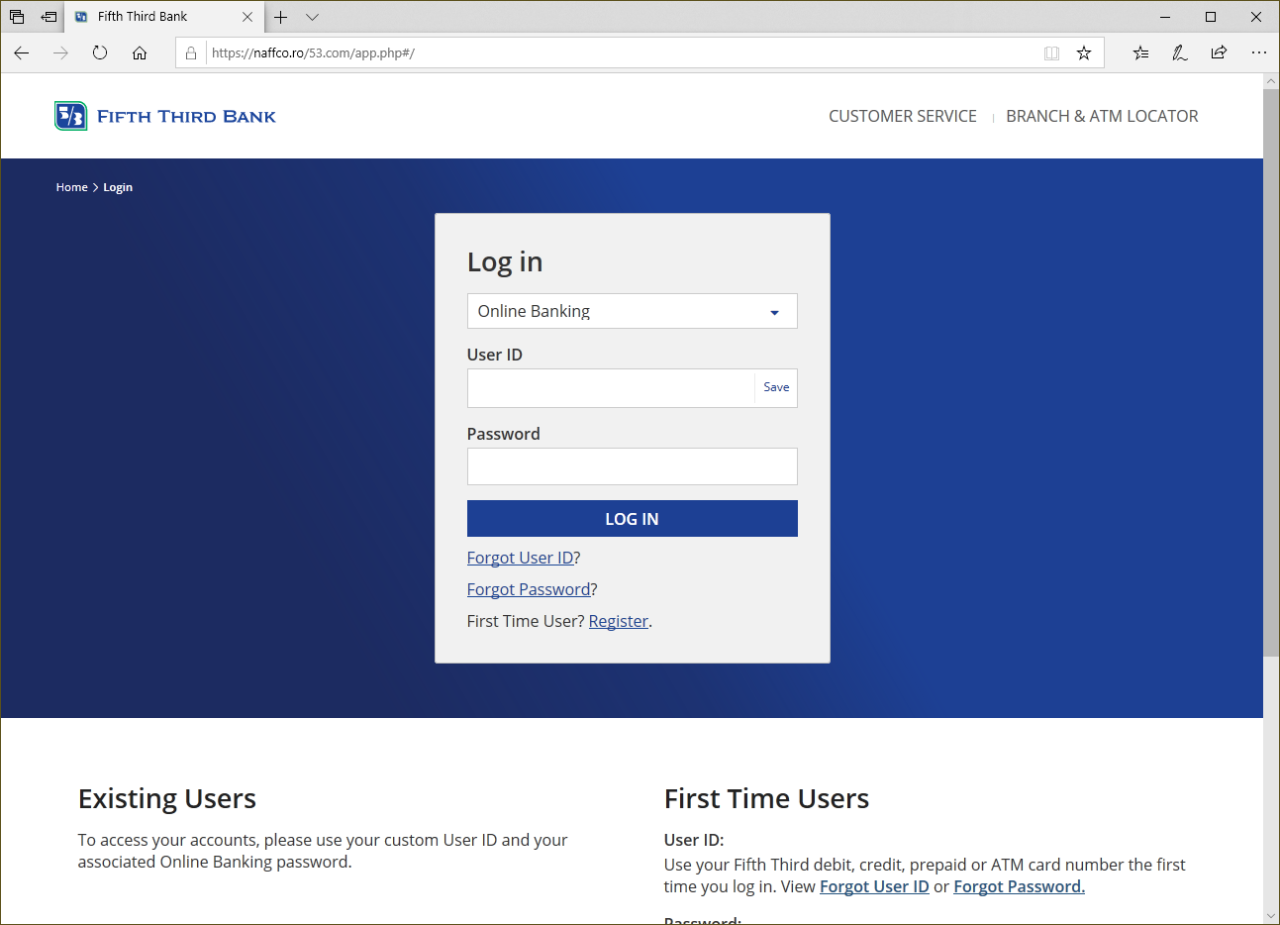This image illustrates the login page of Fifth Third Bank as displayed on a desktop or laptop screen. In the upper left corner of the browser, a tab reads "Fifth Third Bank." Directly below the tab is the address bar, centrally positioned. On the left side of this bar, the Fifth Third Bank logo is visible, featuring a blue square with rounded corners topped with a light blue outline. The interior of the square is a darker blue, containing two white symbols that resemble the letters "FB."

To the right of the logo, "Fifth Third Bank" is written in blue text. Moving further right along the same line, there are two menus: one labeled "Customer Service" and the other "Branch & ATM Locator."

The main part of the page predominantly displays a dark blue background. Centrally located within this background is a white square, serving as the login section. This square prominently displays the word "Login" at the top. Below it, a dropdown menu labeled "Online Banking" is followed by input fields for "User ID" and "Password." A blue button labeled "Log In" is situated beneath these fields. Links for "Forgot User ID," "Forgot Password," and "First-Time User Register" are provided just below the login button.

At the bottom left of the white square, there is text for existing users, instructing, "To access your accounts, please use your custom User ID and your associated online banking password." On the bottom right, the text guides first-time users: "First-time users, use your Fifth Third debit, credit, prepaid, or ATM card number the first time you log in. View Forgot User ID or Forgot Password for assistance."